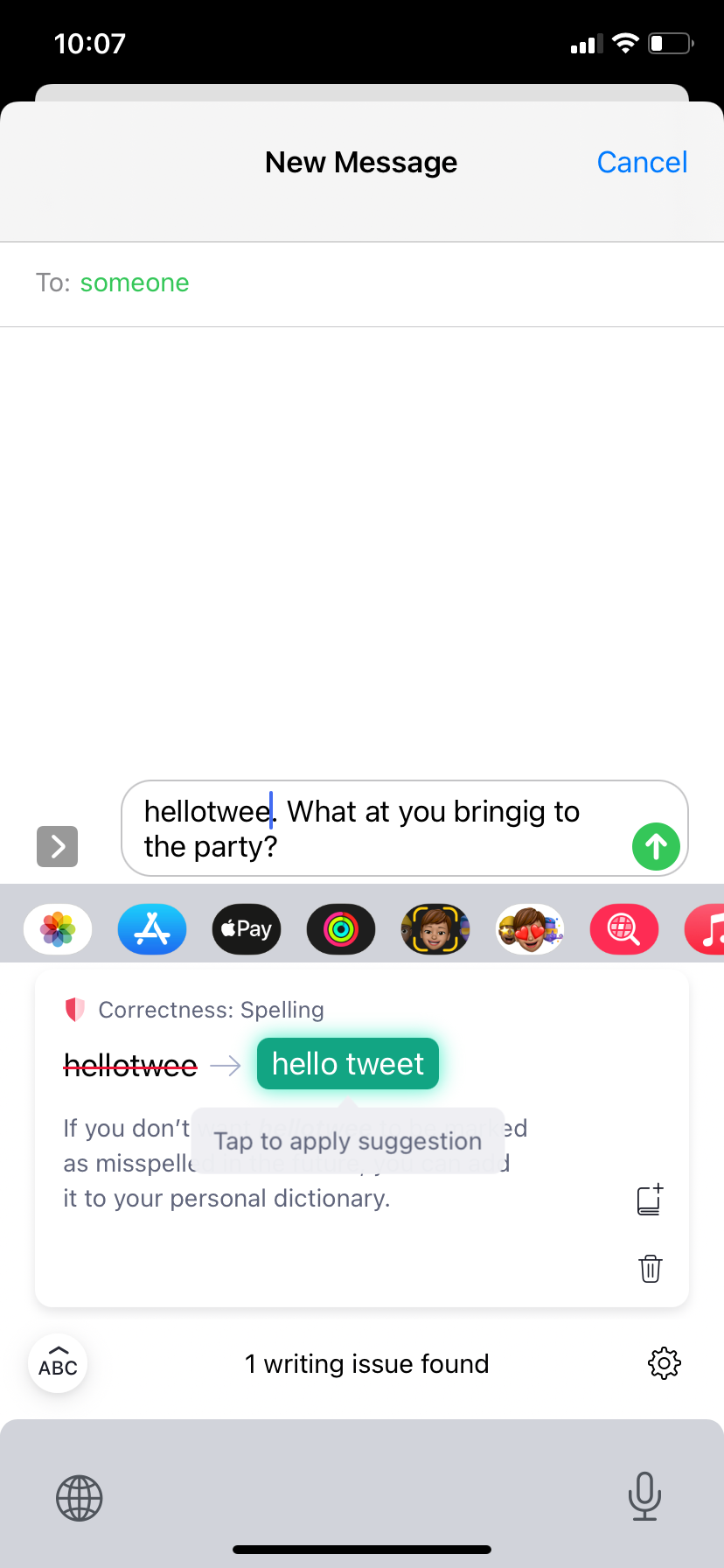This image is a screenshot of an iPhone running iOS, showcasing the iMessages app in the process of composing a new message. At the very top of the screen, a horizontal black bar displays the phone’s status. On the left side of this bar, the current time is shown as "10:07." On the right side, icons indicate the phone’s signal strength, Wi-Fi connection, and battery level, which is approximately one-third full.

Dominating the center is the iMessages interface. At the top, on a gray background, black text reads "New Message." To its right, the word "Cancel" appears in blue text. Just below, a white bar holds the "To:" field, where the placeholder "Someone" is displayed in green text, indicating where a recipient's name or phone number would normally appear.

In the central part of the screen, a gray box outlines the message composition area. Inside this white box, the message reads: "Hello Twee. What at you bring gig to the party?" This text contains several spelling errors. To the right of the message box, a green circle with an upward-pointing arrow serves as the send button.

Beneath the message composition box is a horizontal toolbar featuring various icons, including those for Google Pay and the App Store, showing additional options for the message. Directly below this toolbar, spell check is active and suggests correcting "Hello Twee" to "Hello Tweet." A notification in black text at the bottom of the image states, "One writing issue found," indicating the spell check has identified one error so far.

At the very bottom of the screenshot, from left to right, there is a globe icon for changing the keyboard language, an ABC icon with an arrow in a white circle outlined in gray for the keyboard, a microphone icon for voice input, and a gear icon to access the settings of the Messages app.